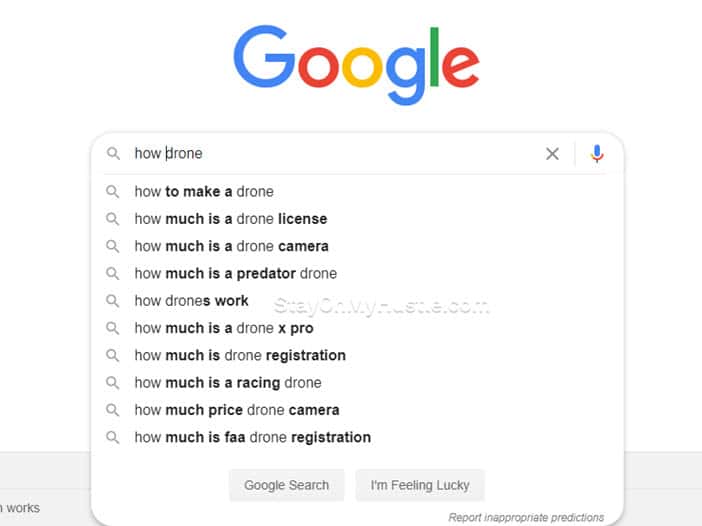This image captures a Google search screen on a typical Windows interface. In the search bar, the user has typed "how drone," prompting a dropdown list of Google search suggestions. These suggestions include queries such as "how to make a drone," "how much is a drone license," "how much is a drone camera," "how much is a Predator drone," "how the drones work," "how much is a drone X-Pro," "how much is drone registration," "how much is a racing drone," "how much price drone camera," and "how much is FAA drone registration." Adjacent to the search bar on the right side is a microphone icon, indicating the option to use voice input for conducting searches.